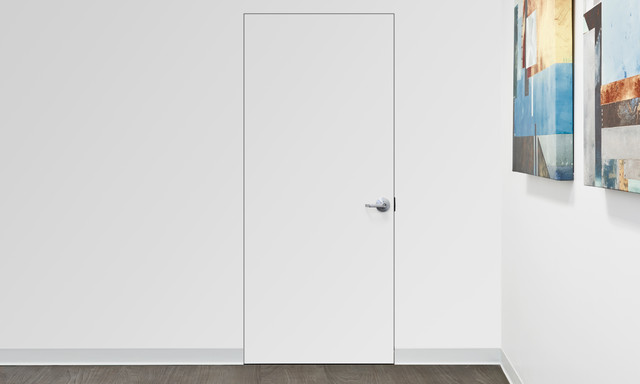This image showcases a minimalist interior with clean, modern design elements. Dominating the scene is a white door that blends almost seamlessly into the adjacent white walls. The door is identifiable primarily by its nickel handle, which has a subtle outline almost directly in the center of the image. The door handle, while silver, merges with the wall’s color, making it nearly invisible at first glance. 

To the right of the door, a vertically-oriented white wall extends towards the viewer, adorned with two pieces of modern abstract art. These artworks feature a mix of blue and brown hues, displayed in various stripes and shapes. The paintings have a three-dimensional quality, with the colorful patterns wrapping around the edges of each canvas. 

At the bottom of the walls, there is a drawn-on dark gray trim that adds a touch of contrast to the light-colored surfaces. The flooring is a rich, dark brown wood, visible at the very edge of the image, grounding the space with warmth and depth. The trim and floor work together to subtly highlight the room's simple yet sophisticated aesthetic.